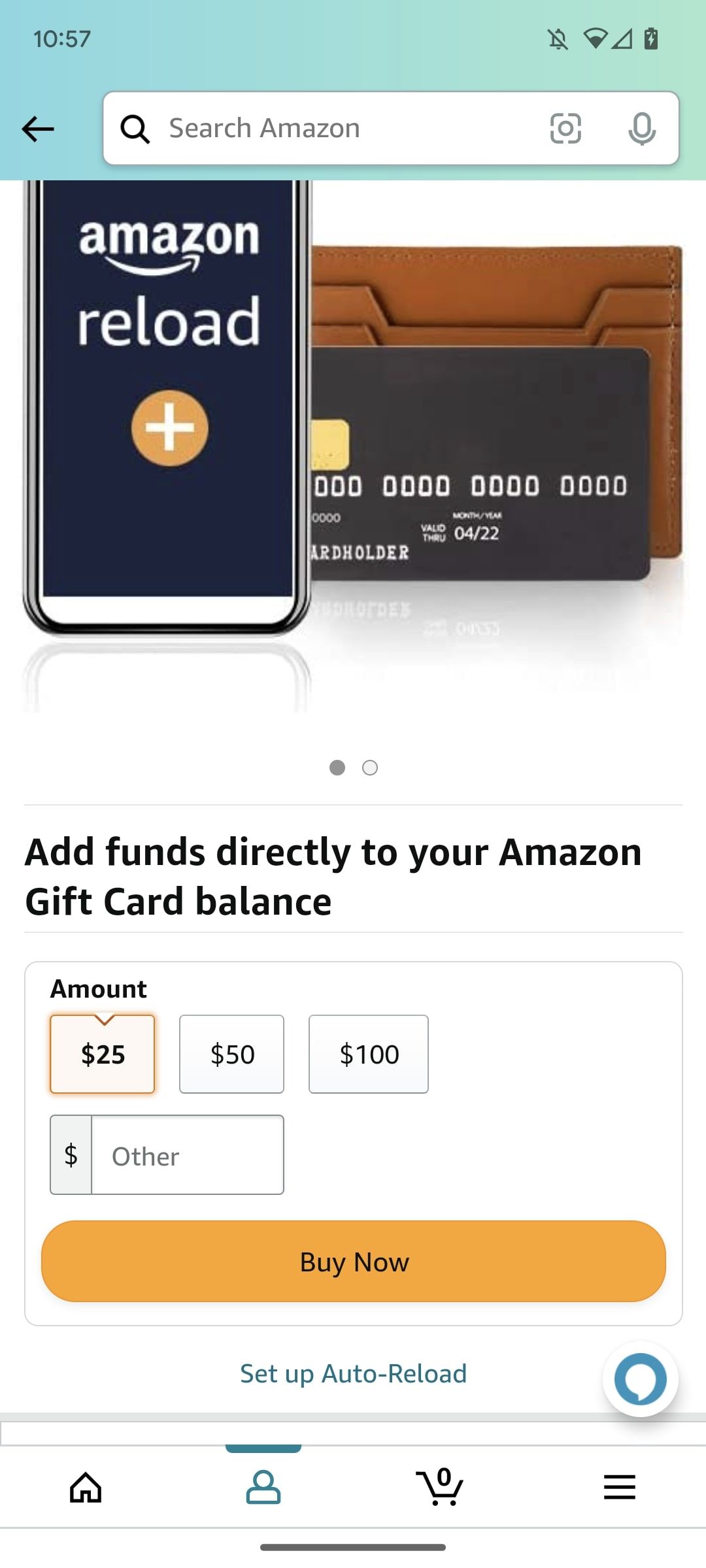The image is a screenshot taken from either a tablet or cell phone, displaying the Amazon Reload page. In the top-right corner of the screen, the time is shown as 10:57. Various icons are visible, indicating notifications are off (denoted by a notification symbol with a line through it), WiFi connectivity, mobile data signal strength, and a nearly full battery.

Occupying the main section of the screen is the Amazon Reload interface. A graphic of a tablet labeled "Amazon Reload" is prominently displayed. To the right of this graphic, there is an illustration of a credit or debit card featuring placeholder information: "Cardholder" and "0000 0000 0000 0000". Positioned behind the card is an image of a wallet.

Below these visuals, text reads "Add funds directly to your Amazon gift card balance". Several preset funding options are provided, with the $25 option currently highlighted. Other visible options include $50 and $100, alongside an "Other" field for entering a custom amount.

Further down, there are prominent buttons labeled "Buy Now" and "Set Up Auto Reload". Additional navigation buttons include "Chat", "Home", "Cart", and a menu button represented by three horizontal lines. The background of the page is predominantly white, and the top section features a search bar labeled "Search Amazon".